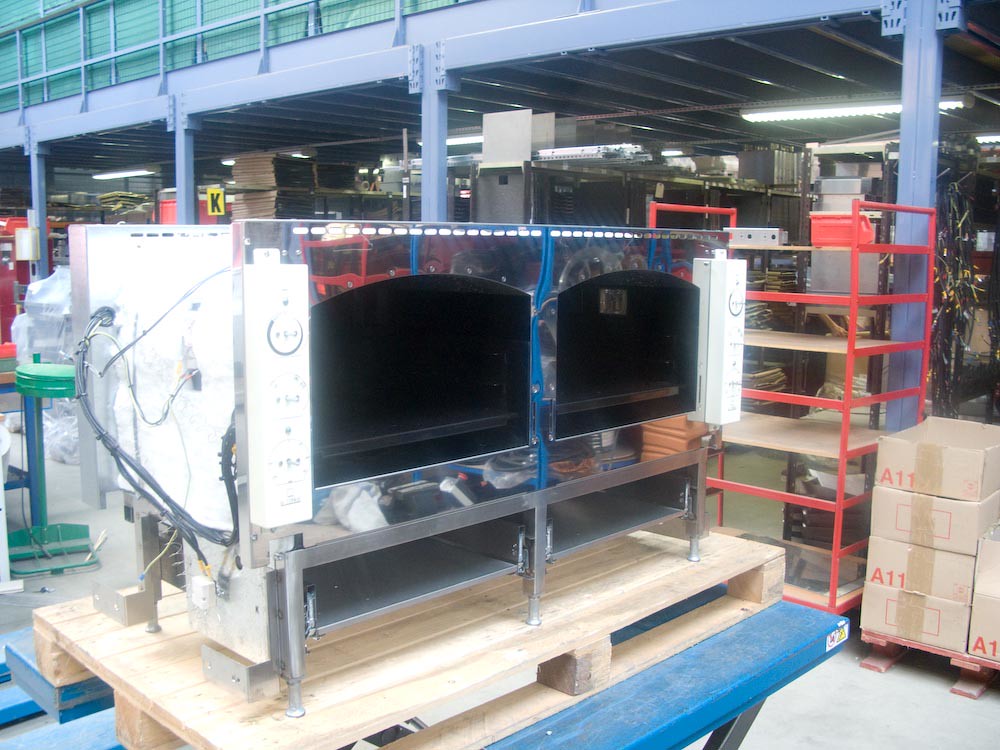This image depicts an industrial factory or machine shop with various storage and workspace areas visible. Prominently in the center front, there is a brown wooden pallet resting on a sturdy blue table with dark gray legs. On top of the pallet sits a large metallic structure resembling a double oven, distinguished by its silver exterior and black interior. The ovens feature white markings on their front panels along with buttons and mechanisms on the side, suggesting they are brand new and potentially used in a restaurant setting. The absence of doors reveals potential racks inside the ovens. To the right of the ovens is an orange rack with brown wooden shelves, and adjacent to it, stacked on a red panel, are several taped-up cardboard boxes labeled "A1." Behind the ovens, a yellow square with the letter "K" is visible, possibly indicating a designated area or safety measure. The upper left section of the image showcases metal beams and a light blue mezzanine with green partitioning, adding to the industrial aesthetic with visible lighting fixtures and absence of a ceiling.